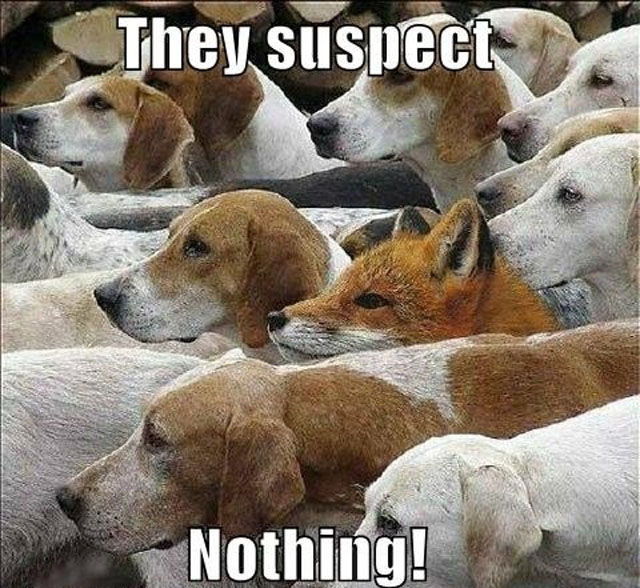This is a square-format meme-style image featuring a large crowd of hunting dogs, primarily beagles and possibly labs, all facing to the left with an intense gaze. They are almost identical in appearance, with predominantly white coats and some exhibiting brown spots. Nestled amidst the sea of canine heads is a conspicuous red fox, characterized by its pointed up ears, white muzzle, black nose, and black-tipped ears, also gazing to the left. The photograph has a realistic, possibly photo-manipulated aesthetic, typical of meme-style imagery. The text at the top in bold white font with a black outline reads, "They Suspect!" while the bottom text says, "Nothing!" Both phrases use an impact font with specific capitalizations, adding to the meme's humor.